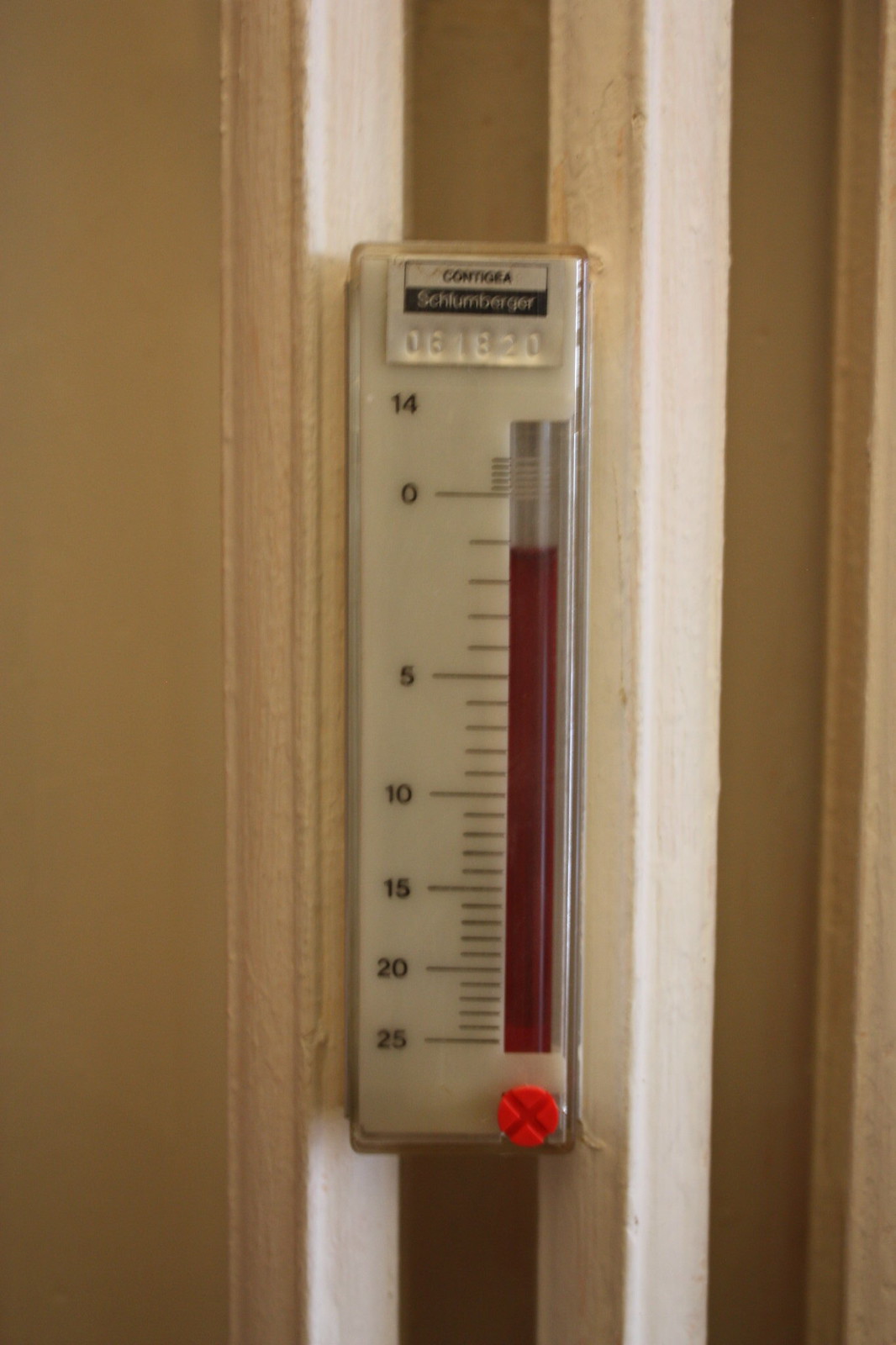The image depicts a detailed thermometer with a rectangular shape, primarily white in color. It stands tall, with a distinctive red circle featuring an X mark located in the bottom right corner. Extending upwards from this circle, a cylindrical tube filled partially with a red liquid is visible. The liquid level reaches near the upper lines but does not fill the cylinder entirely.

Adjacent to the liquid column, a graduated scale with numerical markings can be seen. The scale starts at the bottom with the number 25, followed by descending increments: 20, 15, 10, 5, and zero. Opposite this, at the top of the thermometer, the number 14 is displayed.

Above this, there is a small rectangular section labeled "Contigia" and a text string that reads "S-C-H-L-U-M-B-E-R-D-E-R." Additionally, it features a numeric sequence which appears to be "061821" or possibly "061820."

The background of the image is also white, suggesting the thermometer is mounted on a wall or fitted into a groove on a wall. The structure around the thermometer has segments that protrude slightly, with flatter areas in the background, providing a distinctive and secure placement for the device.